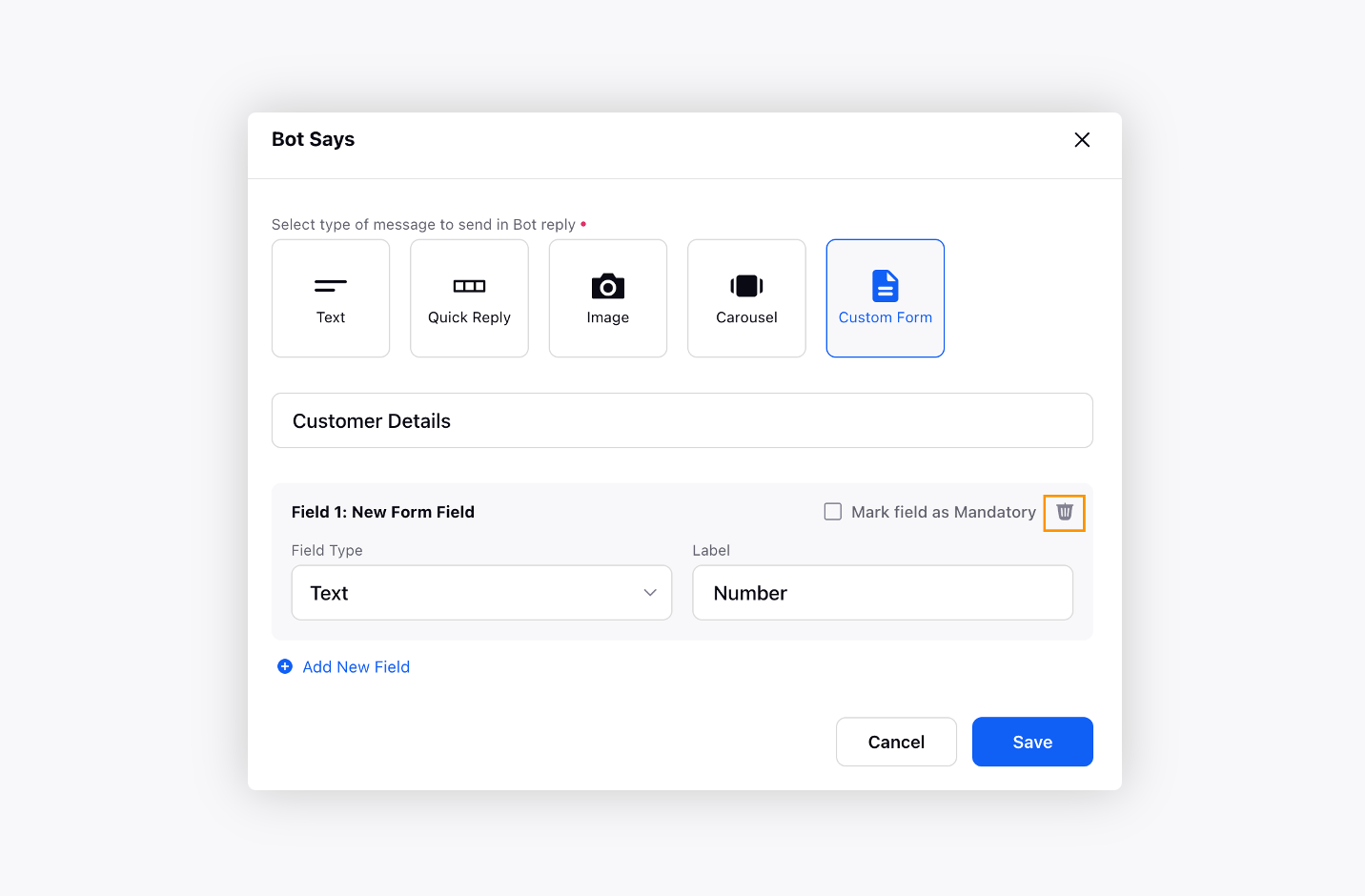The image showcases a user interface on a digital platform, primarily focused on setting up various types of messages for a bot. In the upper left-hand corner, there is a white box containing the text "bot says" in black lettering. To the far right of this box is a black 'X' icon.

Below this, a section allows users to select the type of message to send to the bot, indicated by the phrase "select type of message to send to bot" accompanied by a red asterisk. Underneath are options:

1. **Text**: Represented by two lines of varying lengths.
2. **Quick Reply**: Illustrated by three interconnected squares.
3. **Image**: Symbolized by a camera icon within a square.
4. **Carousel**: Depicted as a more square, football-like shape.
5. **Custom Form**: Shown as a blue piece of paper with a white folded corner, featuring two white lines in the middle.

The highlighted blue box underneath the options is labeled "customer details" in black lettering. Here, there is another box with a gray background and black text that reads "field one, new form field."

To the right of this box, a gray section contains the text "mark field as mandatory," accompanied by an orange square featuring a garbage can icon.

Further below, details for configuring fields are visible. The fields are labeled:
- "Field type" followed by a drop-down box displaying "text" with an arrow pointing down.
- "Number" is listed next to this.

In the bottom left corner, a blue circle with a plus sign and the text "add new field" in blue lettering invite users to add fields. There are also "cancel" and "save" buttons at the bottom: the "cancel" button has a white background with black lettering, while the "save" button features a blue background with white lettering.